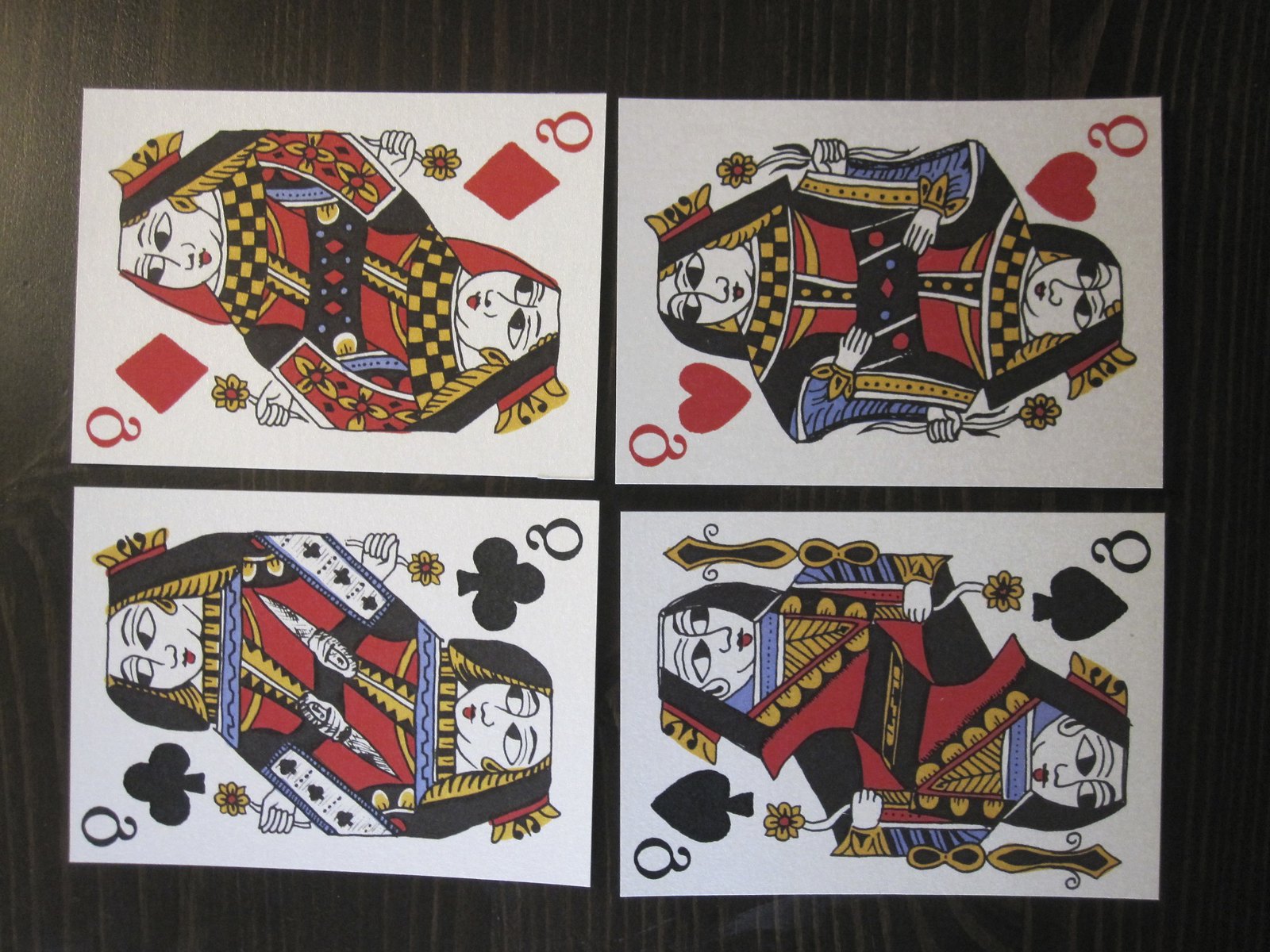The image features four cartoonish flying cars, each designed to resemble a queen from a deck of cards, specifically one of each suit: spade, diamond, heart, and club. The queens are oriented sideways, giving an unusual perspective to the scene. These queens retain the traditional playing card design but are rendered with a lively, animated twist. Notably, the Queen of Spades and possibly the Queen of Clubs appear to have their tongues slightly sticking out, though it could just be a peculiar depiction of their lips. The cards are symmetrically arranged, so the image maintains its orientation regardless of the angle at which it's viewed.